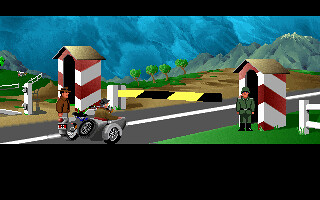The image appears to be a screenshot from a computer game. It depicts a detailed scene at a military checkpoint. In the foreground, a grey road with a white line down its center leads into the distance, blocked by a yellow and black striped barrier. On either side of the road are two small red and white cabins with roofs, resembling candy cane stripes. A soldier in a green uniform stands outside the right cabin, which is situated on green grass, while the left cabin sits on brown dirt.

Next to the barrier is a motorcycle with a sidecar. The driver, on the left, wears a brown jacket and stands beside the motorcycle. The passenger, seated in the sidecar, also dons a brown jacket, albeit lighter in shade. A spare tire is visible behind the passenger seat.

In the distance, the landscape features a range of grey and blue mountain tops, green trees, and stretches of brown soil. The image is presented within a game screen, distinguished by black bars at the top and bottom, with the bottom bar being significantly larger. The entire scene exudes a cartoonish, yet detailed atmosphere, characteristic of video game visuals.